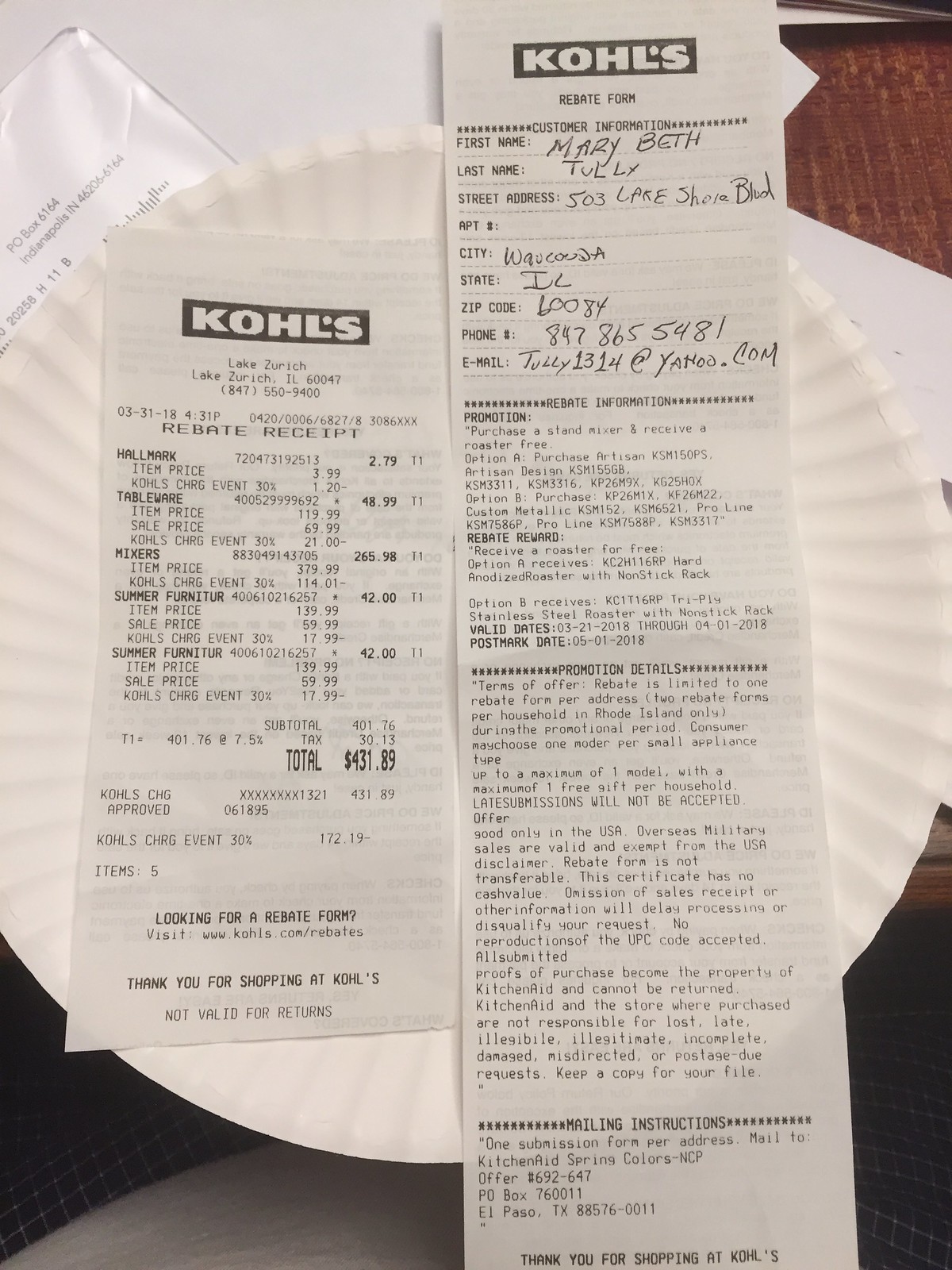The image is a close-up of two Kohl's receipts placed on a white paper plate, which rests on a table. In the top left corner, part of the person's mail is partially visible, slightly cut off by the edge of the frame. The receipt on the left is from Kohl's, originating from Lake Zurich, Illinois, detailing several purchases that total $431.89. The second receipt, to the right, is a completed Kohl's rebate form ready to be mailed. The meticulous arrangement suggests the individual is preparing to send in the necessary documentation to claim their rebate.